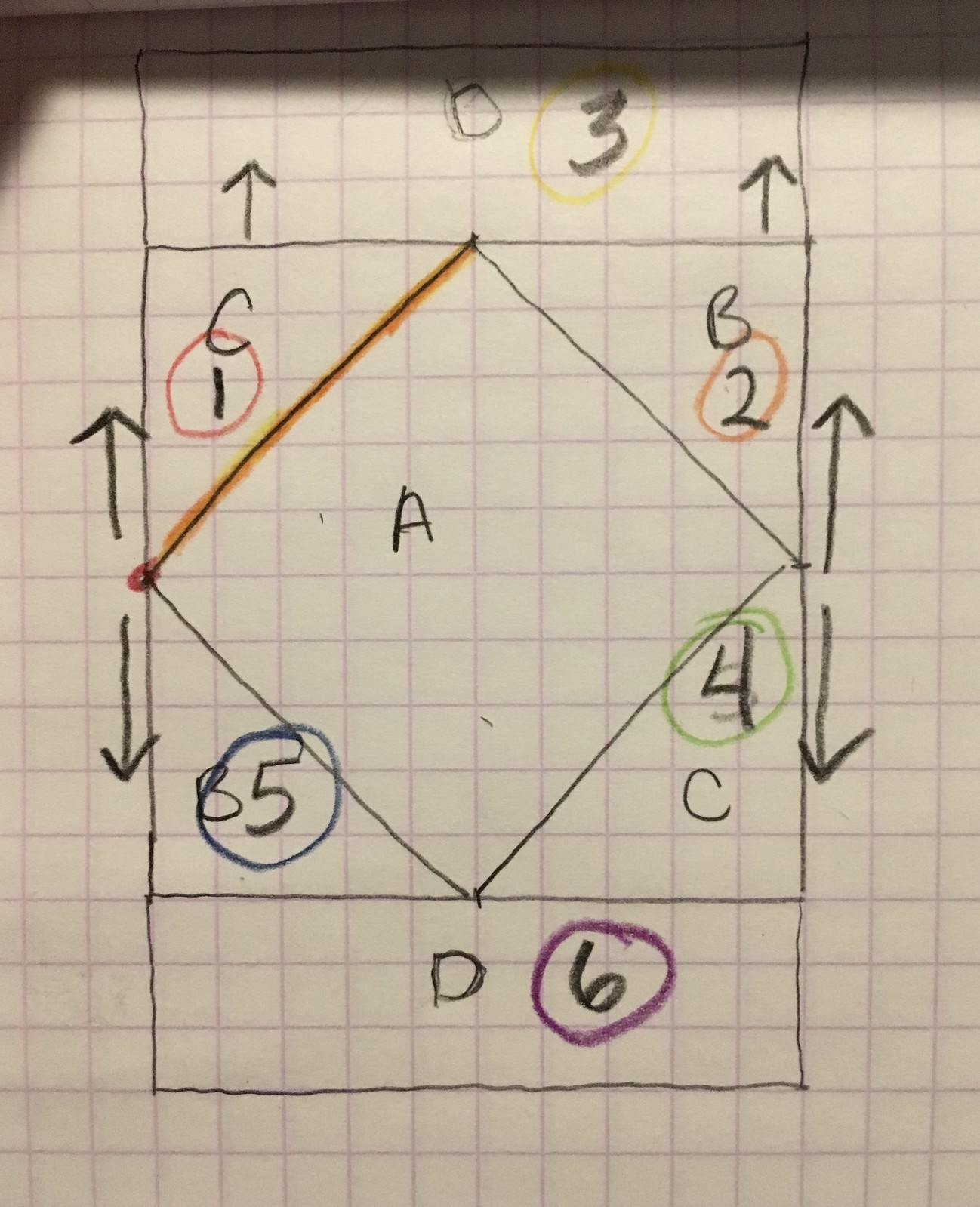This is a detailed overhead photograph of graph paper featuring a range of geometric shapes and annotated elements. 

At the center of the graph paper, there is a diamond shape with the letter "A" positioned slightly off-center to the left and upward within the diamond. Surrounding the diamond, a square frame is drawn, creating four triangular sections at each corner of the diamond. 

In the top left triangle, the letter "C" is located, with the number "1" below it, circled in red. In the top right triangle, the letter "B" is present, with the number "2" beneath it, circled in orange. In the bottom right triangle, the number "4" is circled in green with the letter "C" below it. The bottom left triangle features the number "5" circled in blue, with the letter "B" beside it.

Extending downward from the square is a rectangle with the letter "D" in the middle and the number "6" slightly off to the right, circled in purple. A second rectangle extends upward from the square, also containing the letter "D" in the middle and the number "3" to the side, circled in yellow. This upper rectangle also features arrows pointing upward on both the left and right sides.

Additionally, the original square has arrows pointing upward and downward from the middle on both the left and right sides, positioned just outside the square's boundary. 

Furthermore, the image includes an additional rectangle with three numbers inside and one number outside, giving the structure an architectural appearance reminiscent of a church flanked by houses. This secondary rectangle appears to feature detailed annotations, though not perfectly clear in this description, hinting at complex relationships or diagrams within the shape.

Overall, the annotated shapes and their interconnected elements create a visually intricate and information-rich arrangement on the graph paper.